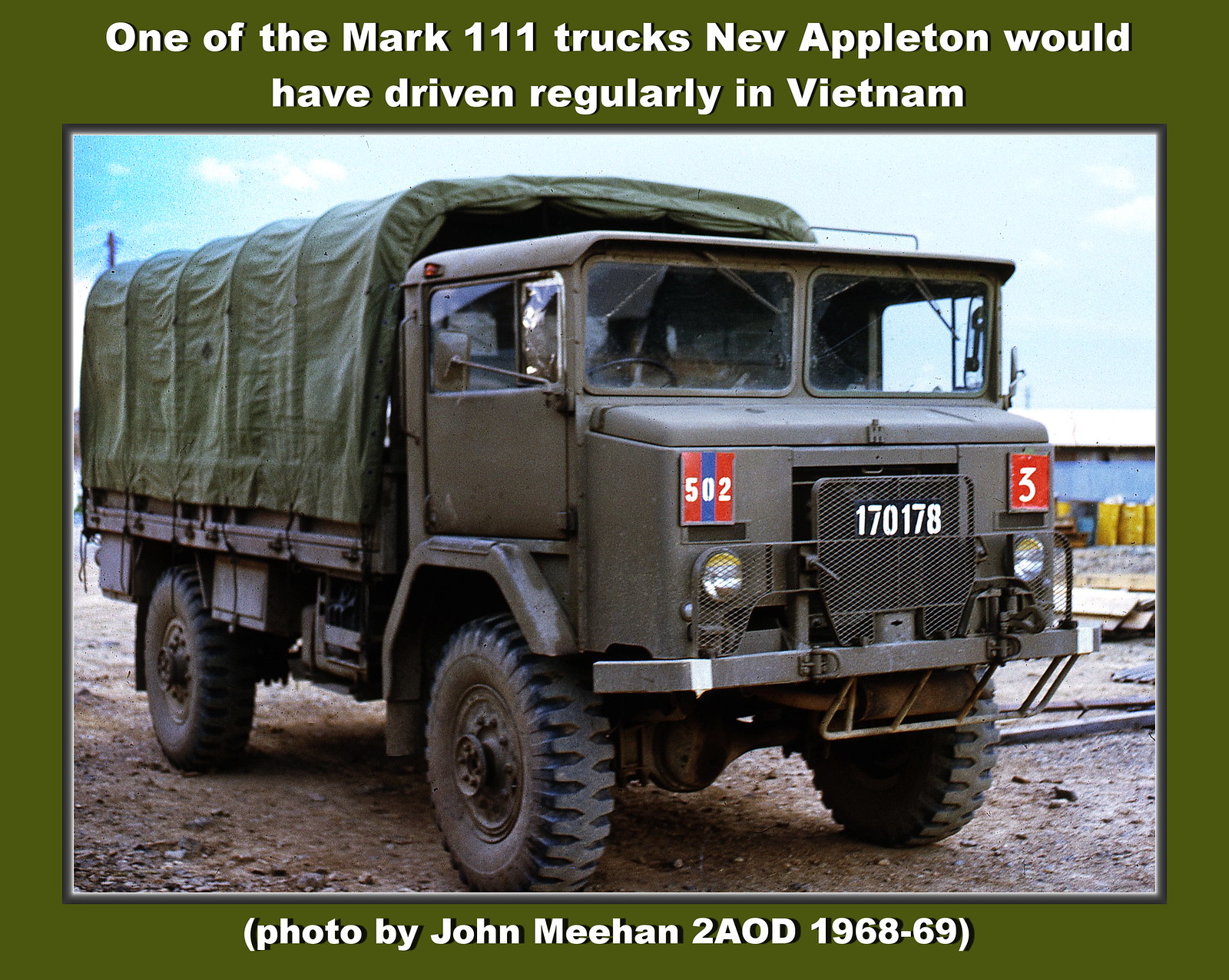The image shows a gray Mark 111 military truck that Nev Appleton would have driven regularly in Vietnam. The truck, captured in a photo by John Meehan from 2AOD during 1968-69, features large off-road tires and industrial screens protecting the front windows. The truck has a green canopy covering the back and is parked on a dirt road. Above the truck, the sky is visible, and in the distance, there are yellow barrels. The photograph includes printed white lettering at the top and has a green border, enhancing its presentation as a historical military vehicle commonly used during the Vietnam War. The truck bears the number 502 on the front, emphasizing its military utility.